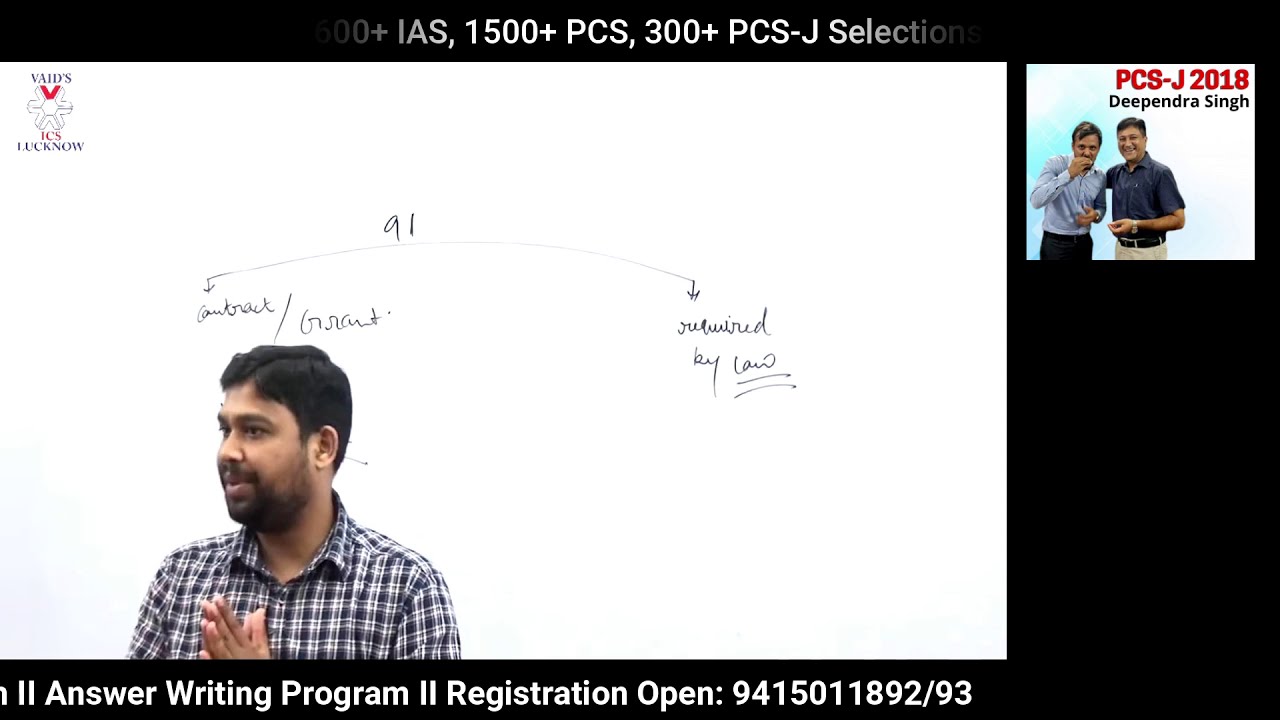The image is an advertisement featuring a man standing in front of a whiteboard, positioned towards the lower left side of the frame. He is a brown-skinned male with short, dark hair and a scruffy beard, wearing a blue and white checkered button-up shirt. The man holds his hands together in a gesture resembling a prayer, with palms pressed, in front of his chest. The whiteboard behind him contains various texts, including the terms "contract grant revised by law," connected by a double arrow, along with the number 91. Additionally, the upper left corner of the image features a small symbol. At the bottom of the image, there is a black strip of text that reads, "Answer Writing Program, Registration Open," followed by the contact number "941-501-1892-93." The man's posture and the surrounding texts suggest that this advertisement is promoting a writing program.